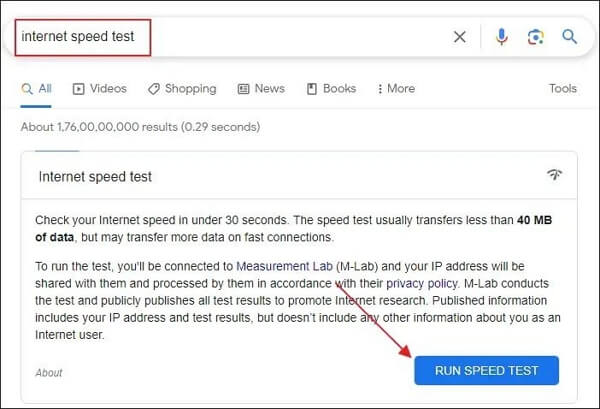This screenshot features a search query interface on a white background with a thin black rectangular border, optimized for a horizontal layout. In the upper left corner, the search box displays "internet speed test," highlighted in red. Adjacent to the search bar on the right are three icons: a Google microphone for voice search, a camera symbol, and a magnifying glass representing the search function.

Directly beneath the search bar, a navigation menu spans from left to right, listing options such as All, Videos, Shopping, News, Books, More, and Tools. Below this menu, there is a brief synopsis indicating that approximately 1,760,000,000 results were generated in 0.29 seconds.

The primary search result centers around the "internet speed test" and provides a brief description: "Check your internet speed in under 30 seconds. The speed test usually transfers less than 40 MB of data but may transfer more data on fast connections." It further explains that running the test will connect the user to Measurement Lab and that their IP address will be shared and processed according to Measurement Lab’s privacy policy.